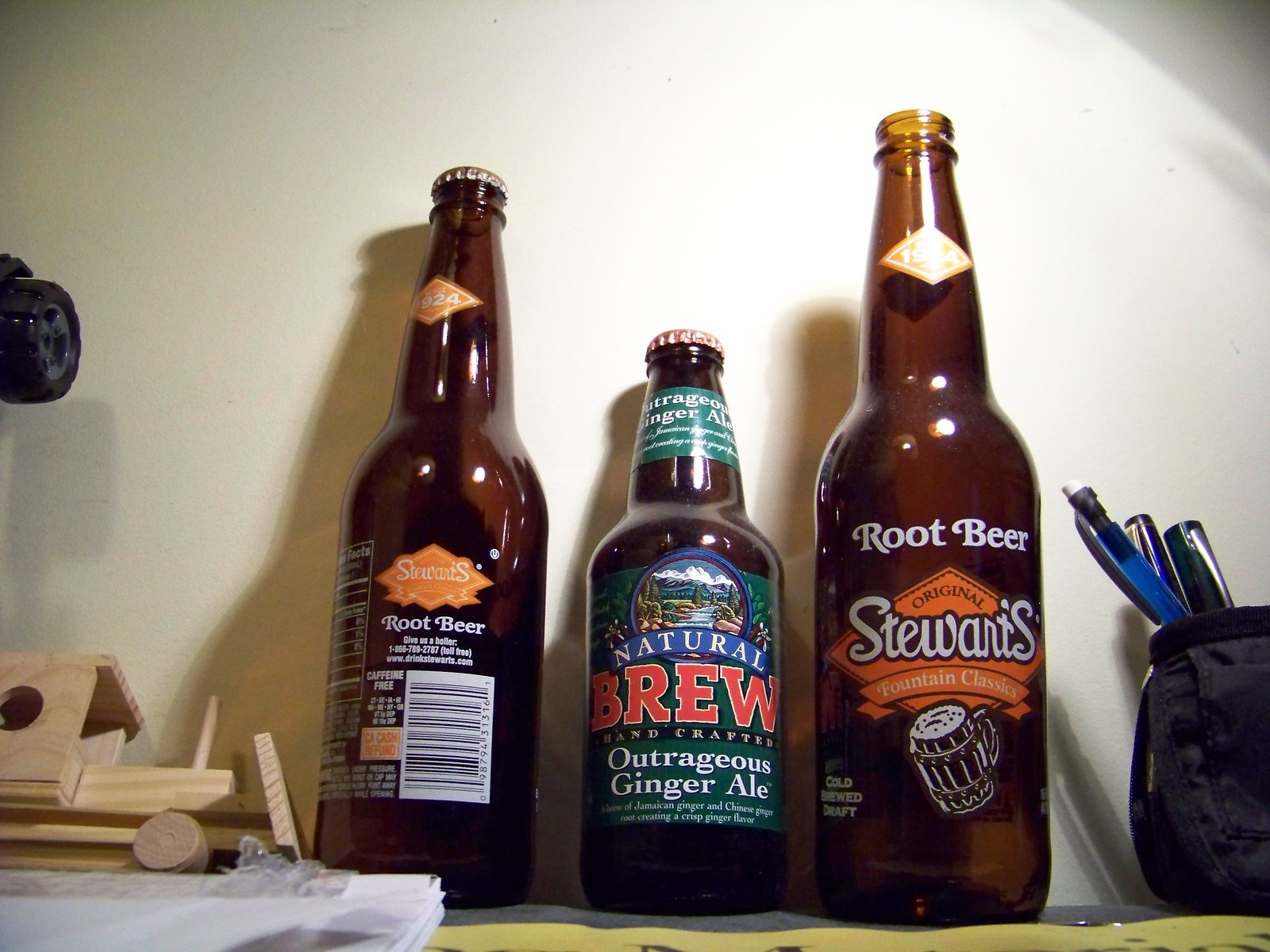The image captures a side-view of three distinct soda bottles arranged on a white-painted shelf, casting light shadows on the background. The first bottle on the left is Stewart's Root Beer with a distinctive brown glass and an orange label adorned with white writing, although its back side is facing us, revealing nutritional information. To its right is a shorter, capped bottle labeled Natural Brew Handcrafted Outrageous Ginger Ale, with a green label featuring red and white text. The third bottle, positioned on the far right, is another Stewart's Root Beer, identical in its brown glass and orange-and-white label, but this one is uncapped with its front label clearly legible. Adjacent to the bottles, a homemade wooden toy car, reminiscent of a bulldozer, sits on the shelf, alongside a cup filled with jumbo pens and writing utensils. This carefully arranged scene highlights both the unique characteristics of each bottle and the quaint, crafted objects that accompany them.